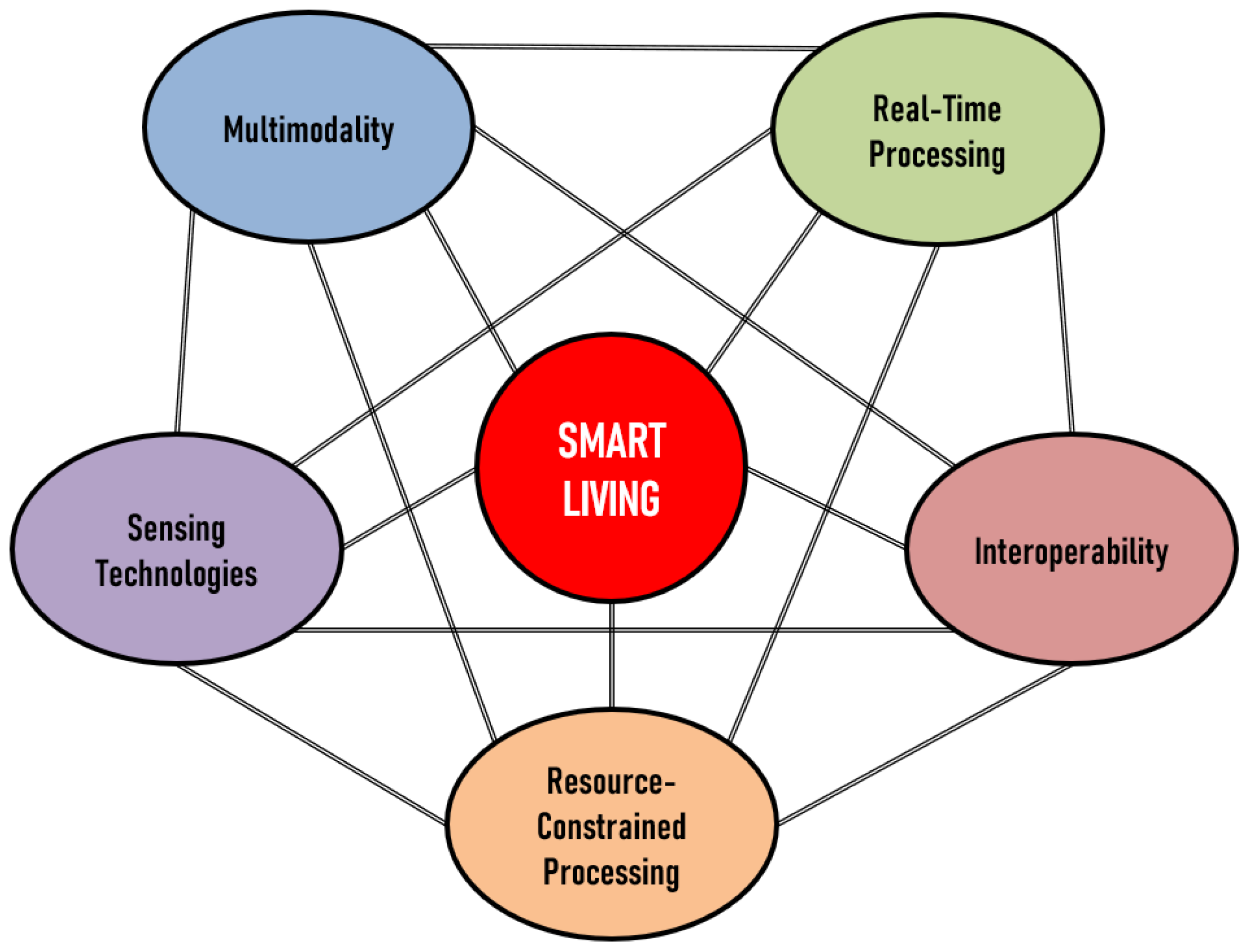The image depicts a schematic diagram on a white background, featuring a central red circle labeled "Smart Living," bordered in black. This circle is interconnected with five colored ovals via lines, representing different categories related to smart living. The ovals and their corresponding colors and labels are: 

- Blue oval labeled "Multi-Modality" (upper left)
- Green oval labeled "Real-Time Processing" (upper right)
- Pink oval labeled "Interoperability" (right-center)
- Orange oval labeled "Resource-Constrained Processing" (bottom)
- Purple oval labeled "Sensing Technology" (center)

These ovals are arranged in a way that they form a network of lines converging towards the central "Smart Living" circle, illustrating the various aspects that make up the concept of smart living.